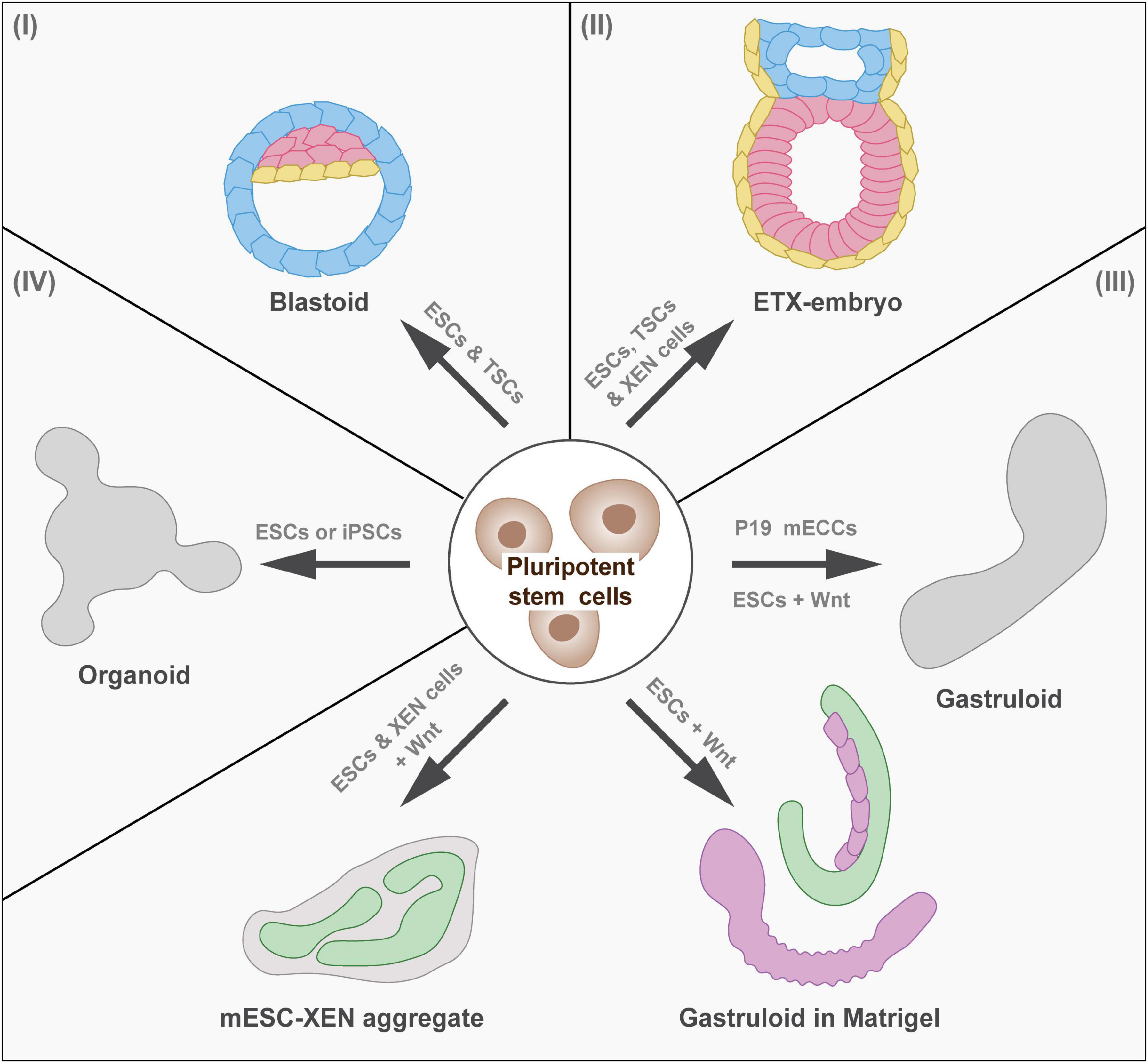This image is a detailed scientific diagram displayed on a white background, likely intended for a presentation or medical textbook. Central to the diagram is a circle labeled "Pluripotent Stem Cells," featuring three brownish circular cells with darker centers. Arrows extend from this central circle to various sections, each highlighting different types of cellular structures with intricate descriptions and labels.

In the upper left section, labeled "1," an arrow labeled "ESCs and TSCs" points to a "Blastoid." This blastoid is depicted with a thick blue segmented outer layer, housing white, yellow, and pink segmented components inside.

To the right, in section "2," an arrow marked "ESCs, TSCs, and XEN cells" directs attention to an "ETX Embryo." This embryo features a yellow segmented outer border. Within it, there is a large pink and white segmented circle, topped with a smaller blue and white segmented horizontal circle.

The bottom right, designated as section "3," is the largest area divided by a diagonal line. This section hosts multiple labeled structures. One arrow labeled "P19 MECCs, ESCs, and WNC" points to a purplish irregular-shaped blob marked "Gastroloid." Another arrow inscribed "ESCs and WNC" directs to a pink worm-like structure alongside a green curled form and another purple segmented component, collectively labeled as "Matrigel." A final arrow in this section labeled "ESCs and XEN cells and WNT" points to a lavender amorphous blob with internal green amorphous shapes, tagged as "MESC XEN Aggregate."

To the left, in section "4," an arrow labeled "ESCs or IPSCs" points to a grayish blob with extensions. This structure is denoted as an "Organoid."

The diagram is meticulously sectioned and numbered, providing a comprehensive visual representation of pluripotent stem cells and their derived structures across different contexts, with significant repeating emphasis on "gastroloid" and "matrigel" in the bottom right section, illustrated with distinct pink, purple, and green blobs.